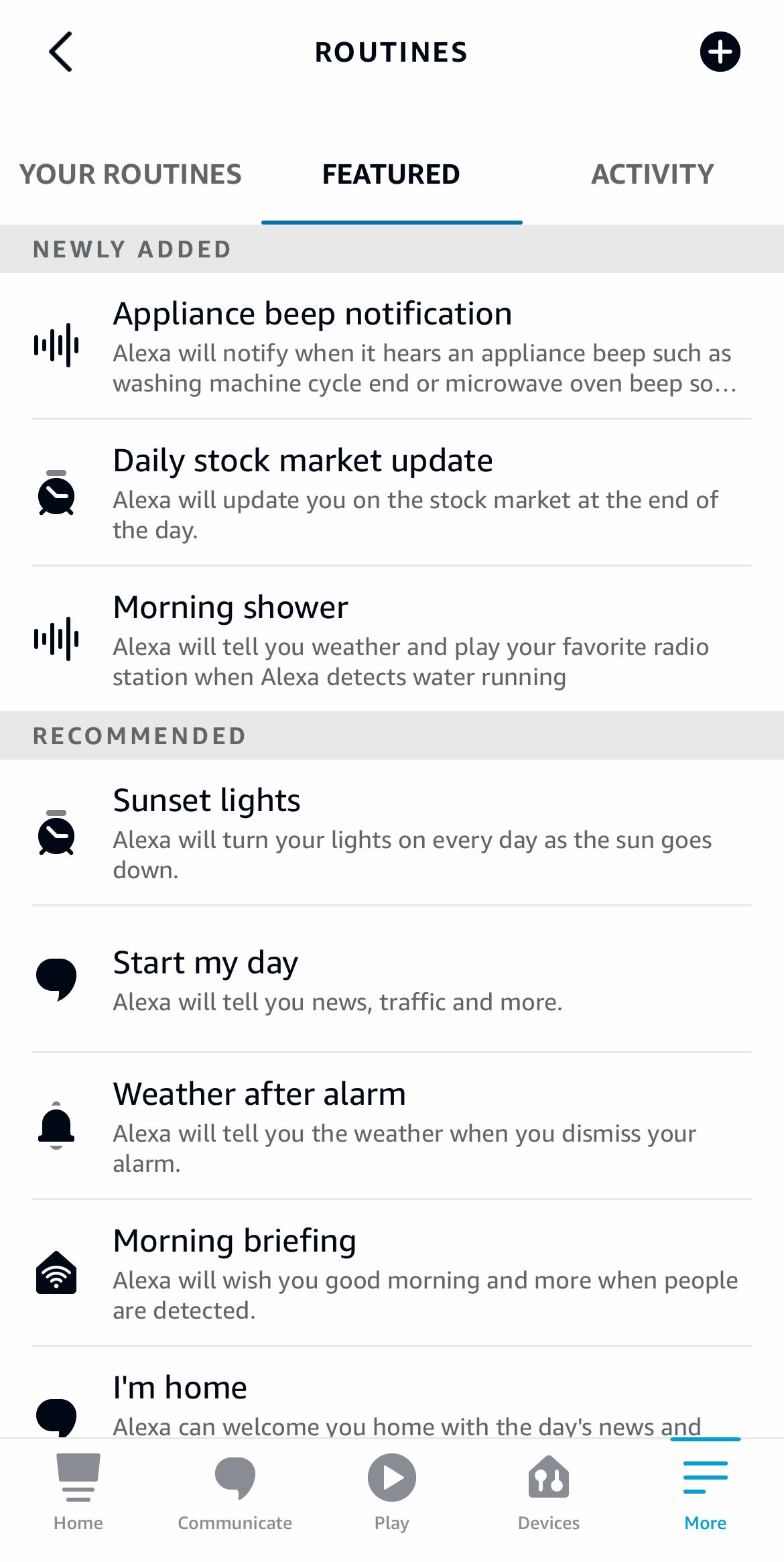This is a detailed screenshot from a mobile phone interface related to routines for Alexa. The background is predominantly white at the top. In the top left corner, there's a small arrow pointing to the left, indicating a back function. Centered at the top is the title "Routines" in bold black font. On the right corner, there's a black circular icon featuring a white plus sign inside it, suggesting an option to add new routines.

Below the top section, in gray font, there's the text "Your Routines." The word "Featured" is prominently displayed in black font with a blue underline indicating it's the selected tab. To its right, "Activity" is marked in gray font, suggesting it’s another available tab.

The section below "Your Routines" is a light gray rectangle with "Newly Added" written in a darker gray font. Under this title, three options are listed:
1. **Appliance Beep Notification** - Alexa will notify you when it detects an appliance beep, such as from a washing machine cycle end or a microwave oven beep. This description is cut off with an ellipsis.
2. **Daily Stock Market Update** - Alexa will provide an update on the stock market at the end of each day.
3. **Morning Shower** - Alexa will announce the weather and play your favorite radio station when it detects water running, ideal for your morning shower.

Following these "Newly Added" routines, there’s another light gray rectangle labeled "Recommended" in darker gray font. The recommended routines listed below include:
1. **Sunset Lights** - Alexa will gradually dim the lights as the sun sets each day.
2. **Start My Day** - Alexa will share the news, traffic updates, and more, likely to kickstart your morning routine effectively.

This detailed screenshot provides a comprehensive look at the available and suggested routines to be set up with Alexa for better daily management and automation.